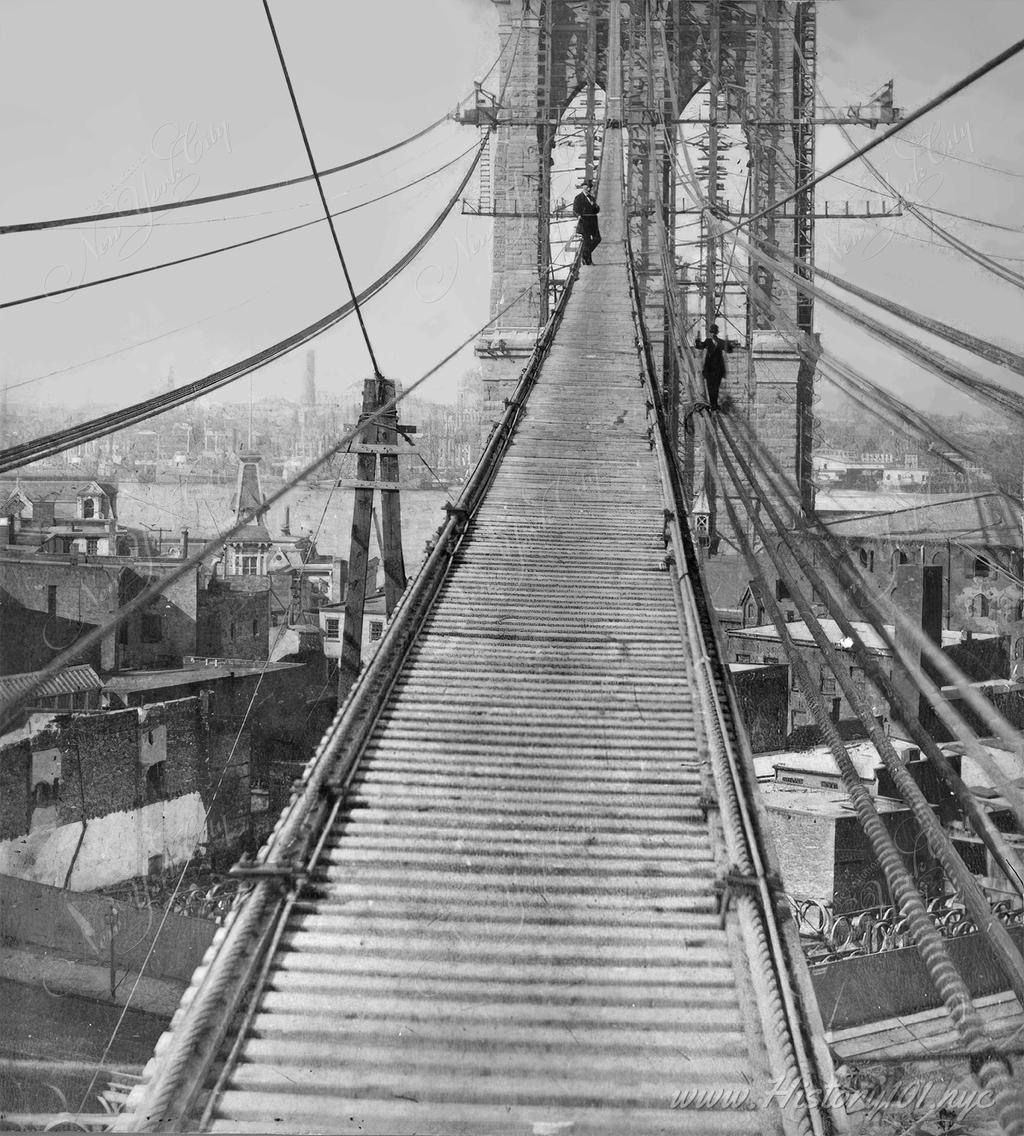This historical black and white photograph captures a striking scene during the construction of the Brooklyn Bridge in New York City, likely taken around a hundred years ago. Prominently featured in the image are two men dressed in suits and top hats, standing casually amidst the bridge’s suspension cables without any protective work gear. The man closer to the camera has his legs crossed and faces the lens, while the other stands further out on the cables, holding something in his hands. Both individuals appear quite composed despite the precarious positions they occupy. Below and beyond the bridge, a cityscape filled with buildings and factories stretches out, with the Hudson River visible further in the background. The distinctive pylon with its double archways, from which numerous cables are suspended, rises majestically amidst the skyline. The image includes the URL www.history101.nyc, indicating its historical significance.